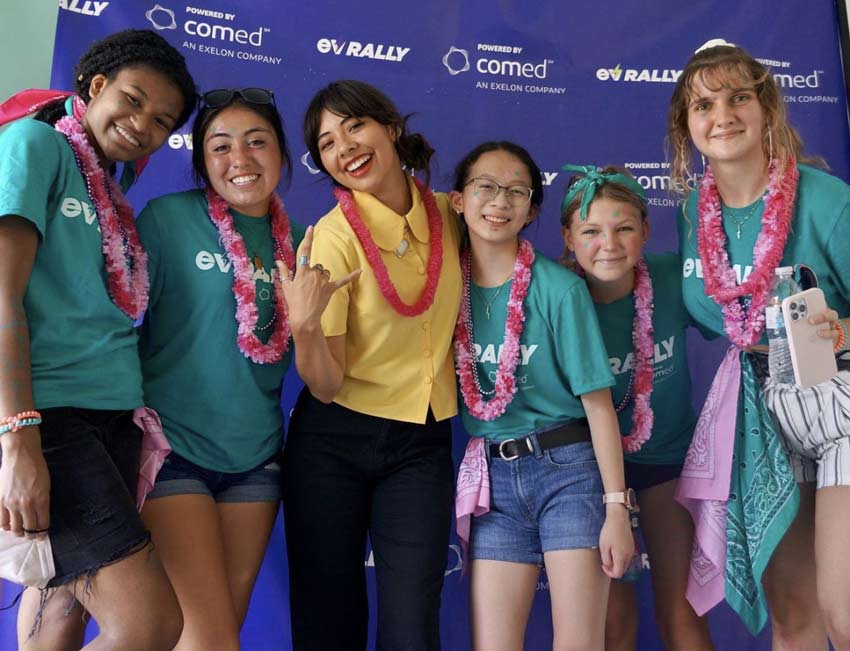The image captures six young ladies attending an event signified by the blue backdrop with white text that reads "ComEd, an Exelon Company" and "EV Rally." From left to right, the first girl is an African-American wearing a pink lei, a green shirt, black cut-off shorts, and two bracelets—one orange, one green—on her wrist. She stands beside a light-complexioned girl, who sports sunglasses perched on her head, a radiant smile, a pink lei, a green shirt, and regular jean shorts. The third individual appears to be an adult, possibly the event organizer, distinguished by her yellow shirt, pink lei, long dark hair, big smile, and blue jeans. Next to her is an Asian girl wearing glasses, a green shirt, blue jeans, and a pink lei. Beside her stands a white girl, slightly squinting, adorned in the same green shirt, pink lei, and a green headband. The last girl, tall with blonde shoulder-length hair, holds a cell phone in one hand and a bottle of water in the other, with two handkerchiefs hanging from her pink lei. All the girls, except the woman in yellow, are under 20, indicating their youthful exuberance at the rally.